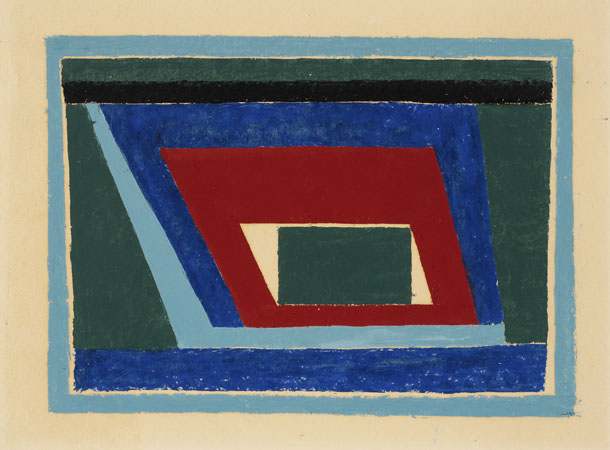The image is an abstract art painting with a background of cream or tan color. At the outermost edge, there's a cream-colored rectangle. Inside this boundary lies a medium blue rectangle. Within this blue rectangle, the inner composition starts with a dark green horizontal bar on top and a black horizontal bar underneath it, followed by a medium blue bar at the bottom. Within these borders, there's a dark teal area.

At the center of the composition, various nested four-sided shapes appear, tilted to the left. From the outermost to the innermost, these shapes begin with light blue, followed by a darker blue, then red, and finally revert to the background cream color or remain empty in the center. At the very core of this nested sequence is a dark green or dark teal small rectangle. The interplay of rectangles, strips, and various geometric shapes creates a dynamic sense of depth and complexity in the artwork.